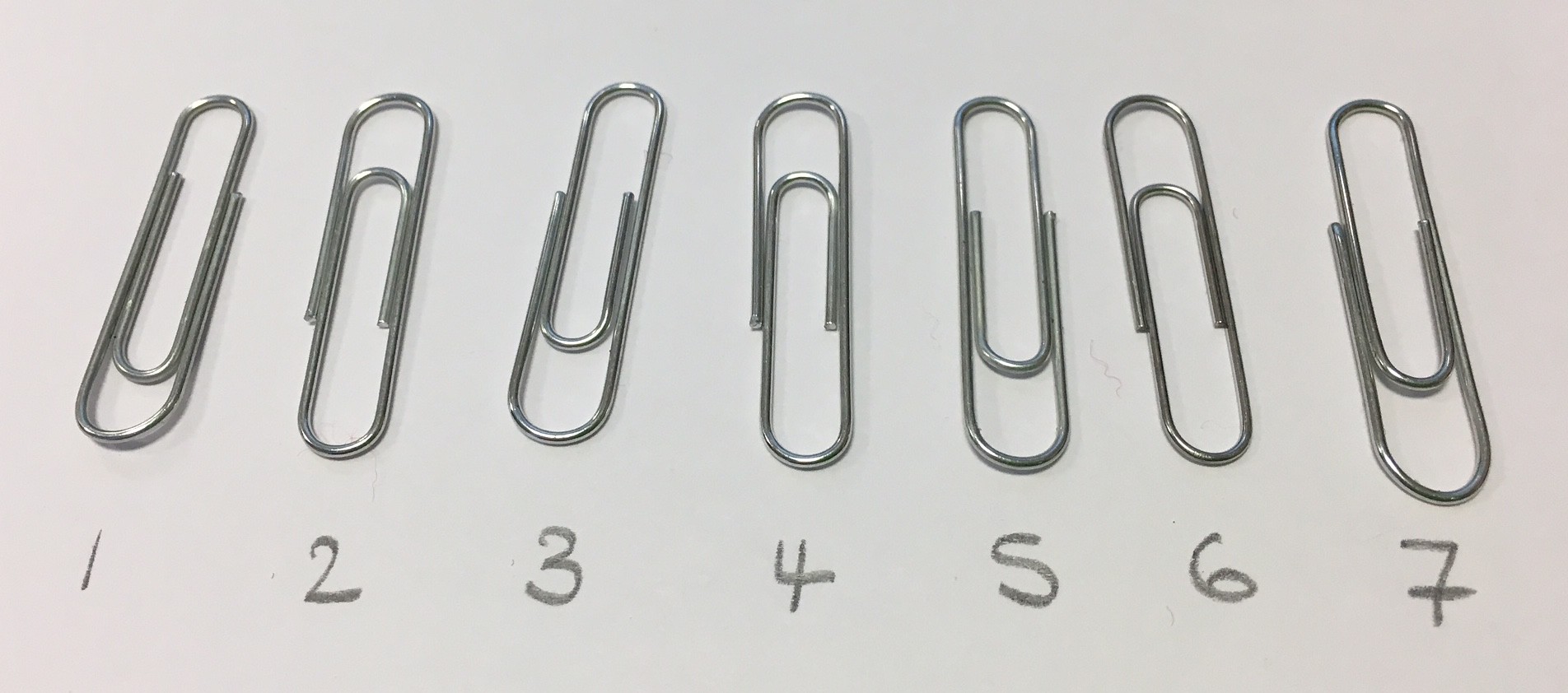This image is a detailed photograph showcasing a neat arrangement of seven paperclips laid out on a piece of white paper. The paperclips are aligned in a single horizontal line from left to right, each labeled with a number beneath it, written in graphite pencil. The numbers start at 1 on the far left and proceed sequentially to 7 on the far right. While all the paperclips are silver and of the classic shape, the one labeled number 7 on the far right appears to be slightly larger than the others. Each paperclip is oriented in the same direction, contributing to the orderly appearance of the display. The background of the photograph is light gray, further highlighting the simplicity and elegance of the white paper and silver paperclips.